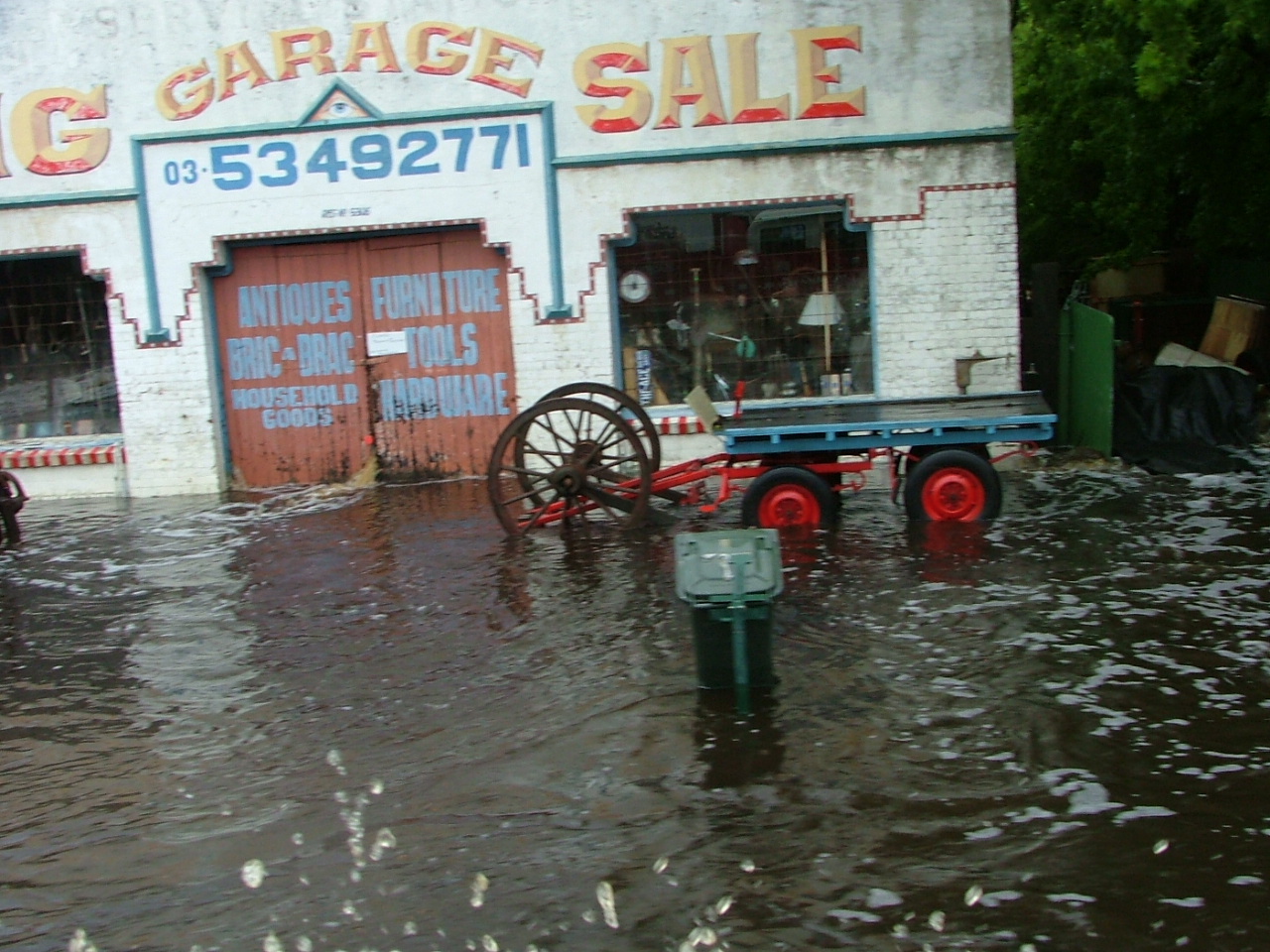The image depicts a white brick building, labeled "Garage Sale" in large orange letters across the top, with a phone number (03-5349-2771) printed below. The entrance features two wooden doors marked with signs for antiques, furniture, brick-a-brack, tools, household goods, and hardware. A single window provides a glimpse inside, revealing various pieces of furniture, such as lamps and clocks. The scene outside the shop showcases significant flooding; water has inundated the front area, creating a semi-submerged landscape. Visible in the water are a trash can and a wheeled carriage or flatbed with four red wheels and two larger rear wheels. Additionally, splashes and droplets rise from the water, suggesting the photograph may have been taken from a low angle or a boat. The street is deserted, with no lights on inside the shop, and nearby, there are pieces of cardboard, wooden trash, and a large tree. The flooding appears to be around eight inches deep, emphasizing the pervasive nature of the floodwaters engulfing the front of this quaint storefront.